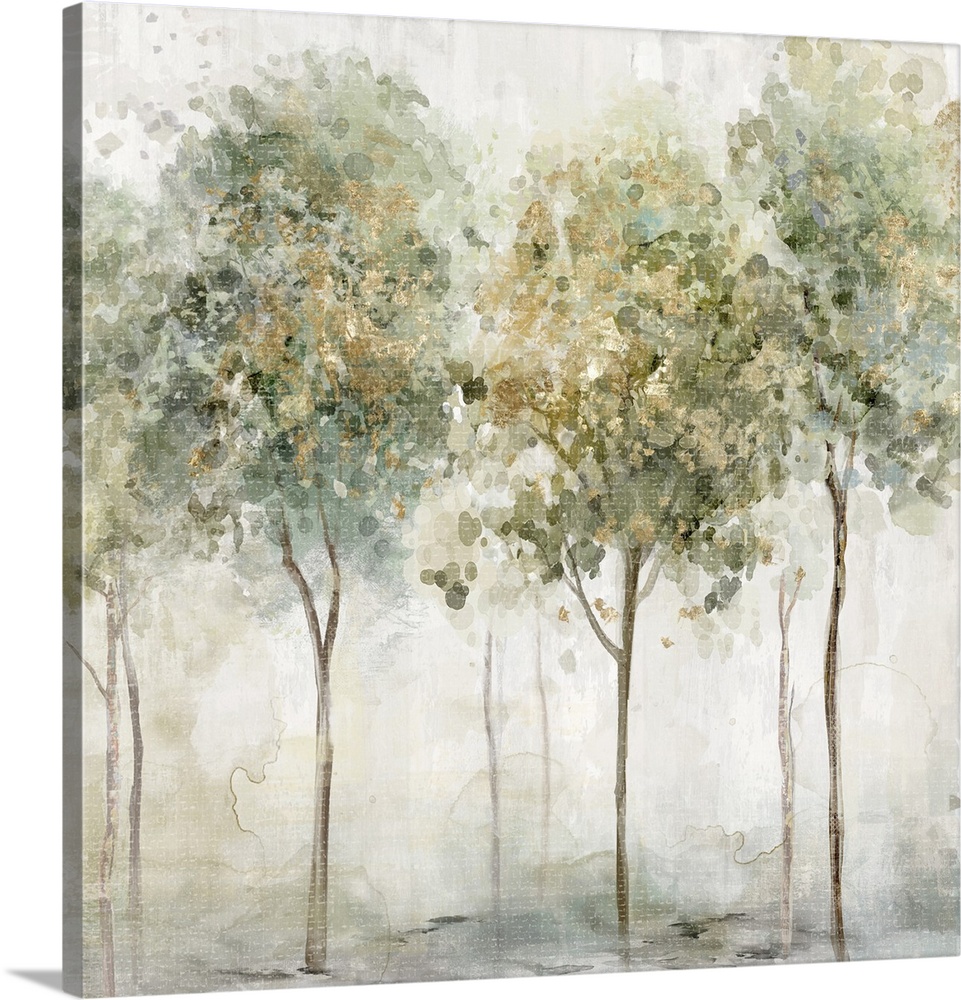This painting, set against an all-white background, vividly captures an abstract depiction of trees on a canvas. The artwork features eight slender trees, though three stand out more distinctly, while others blend into a blurred, foggy backdrop. The trees are adorned with leaves in hues of golden yellow, dark and light greens, blues, and light yellows, creating a lively, splashy effect reminiscent of paint splatters or watercolor blots. The earthy color palette extends to the background, consisting of grays, browns, and subtle yellows, with the watercolors noticeably dried in varied patterns. The tree trunks are brown, and the bottom of the canvas showcases a splattering of grays, blues, and greens, adding depth and texture to the piece. Overall, the painting lacks hard lines, contributing to its dreamlike, abstract quality.